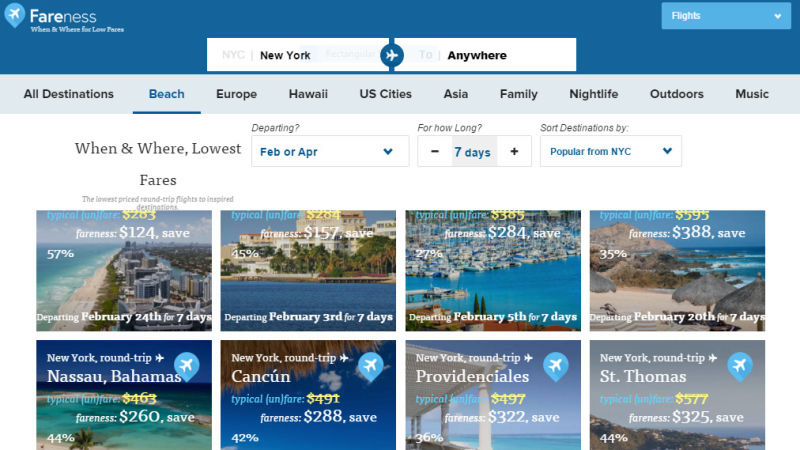The screenshot showcases a travel website. At the top, there is a prominent blue banner featuring an airplane logo within a blue map pin located in the upper left corner. To the right of the logo, the word "Fairness" is displayed in white text. Central to the banner is a white search bar with "New York" on the left side in black text and "Anywhere" on the right. The upper right corner features a blue dropdown box situated above a gray banner.

Below this gray banner, a navigation menu lists various travel categories in black text from left to right, including: "All Destinations," "Beach," "Europe," "Hawaii," "U.S. Cities," "Asia," "Family," "Nightlife," "Outdoors," and "Music." Directly underneath are boxes for selecting a departure date, trip duration, and sorting destinations.

Further down the page, eight vibrant color photographs represent different travel destinations, each presumably linked to more detailed information about the respective location.